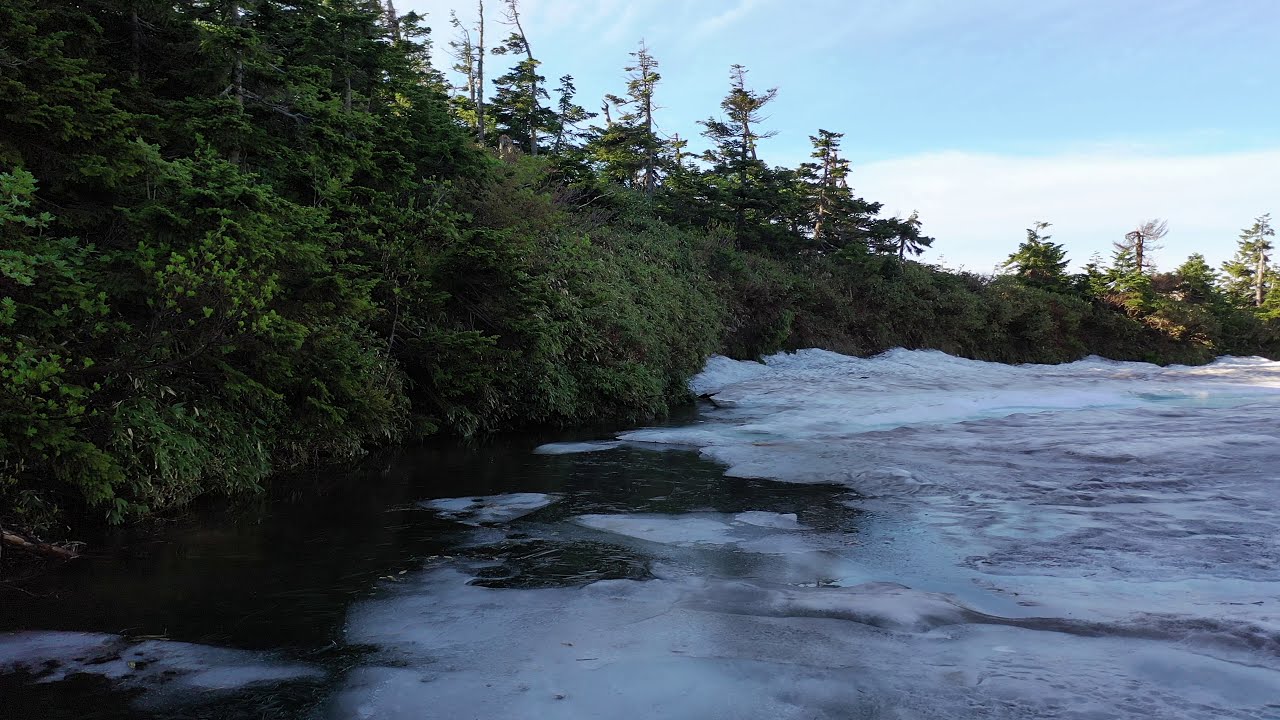In this detailed image, a river or possibly the shoreline of a lake seamlessly blends the elements of winter and early spring or late fall. The bottom half of the image showcases a predominantly frozen river, transitioning from the bottom left to the upper right, with a significant amount of ice covering the right side. The left bank is adorned with lush, green trees and brush that stretch across the entire image, suggesting a transitional season or a colder snap preserving greenery. Patches of thawed water add contrast to the ice, particularly along the left edge near the bank. The vibrant blue sky, dappled with clouds and a hint of sunshine, casts a serene light over the scene, highlighting the peacefulness despite the cold. The overall setting, combined with the natural elements, invites viewers to imagine standing at the water's edge, taking in the crisp air and the picturesque view.